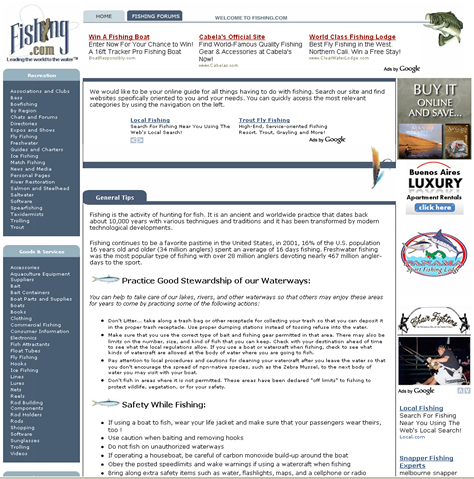**Screenshot Caption: Fishing.com Homepage Overview**

This screenshot captures the homepage of Fishing.com, prominently featuring its banner in the upper right corner, accompanied by what appears to be the tagline: "Leading the Worldwide Fishing Media" (though this text is quite small and difficult to read). The navigational menu includes options like "Home," "Fishing Forums," and a welcome message to the site visitors.

Below the navigation bar, three red headlines catch the viewer's attention with enticing offers: "Win a Fishing Boat," "Cabela's Official Site," and "World-Class Fishing Lodge." On the left side of the image, a graphic showcases a bass fish with its mouth open, seemingly being hooked, adding a dynamic visual to the page.

The right-hand side of the page features two vertical toolbars. The top toolbar is light gray, transitioning to dark blue for the majority of the bars. These toolbars contain numerous options, although their small font makes them hard to decipher. Categories like "Ice Fishing" and "Bow Fishing" are partially visible.

Toward the center-left of the screen, a highlighted text block expresses the site's mission: "We would like to be your online guide for all things having to do with fishing. Search our site and find websites specifically oriented to you and your needs. You can quickly access the most relevant categories by using the navigation on the left." Below this, links to topics such as "A Lot of Fishing" and "Trout Fly Fishing" are available, followed by a general description of fishing that emphasizes its historical and technological evolution.

In the bottom left section, additional links offer enticing opportunities, such as "Buy it Online and Save" and "Buenos Aires Luxury Apartment Rentals."

Overall, this detailed caption provides an overview of the website's content and the layout visible in the screenshot.